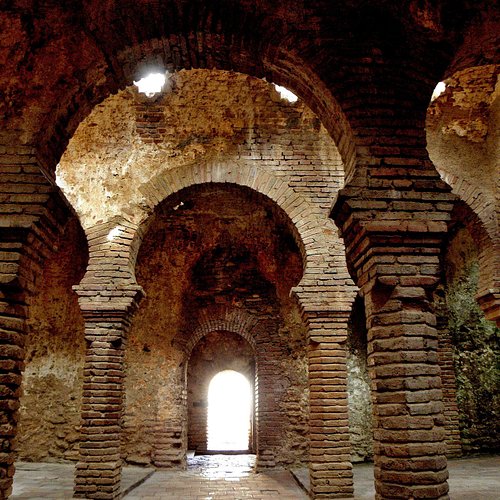This image depicts a remarkably well-preserved ancient ruin characterized by impressive masonry and towering stone arches. The scene is dominated by multiple archways—three of which frame the picture, leading one's eyes to the light streaming in from the entrance. The bricks, a mix of light brown, yellow, tan, red, and rust hues, show signs of extensive wear, hinting at the structure's age and historical significance. The meticulously cut stone columns, some appearing octagonal, add to the ornate complexity of the architecture, while an element of ivy foliage climbs up a wall in the background. Holes near the ceiling allow rays of sunlight to penetrate the space, enhancing the beauty of the scene and emphasizing the grandeur and depth of the structure. This photorealistic capture showcases an architectural marvel from a bygone era, absent of any modern inscriptions or human presence, making the ancient craftsmanship and timeless elegance of the ruins the focal point.